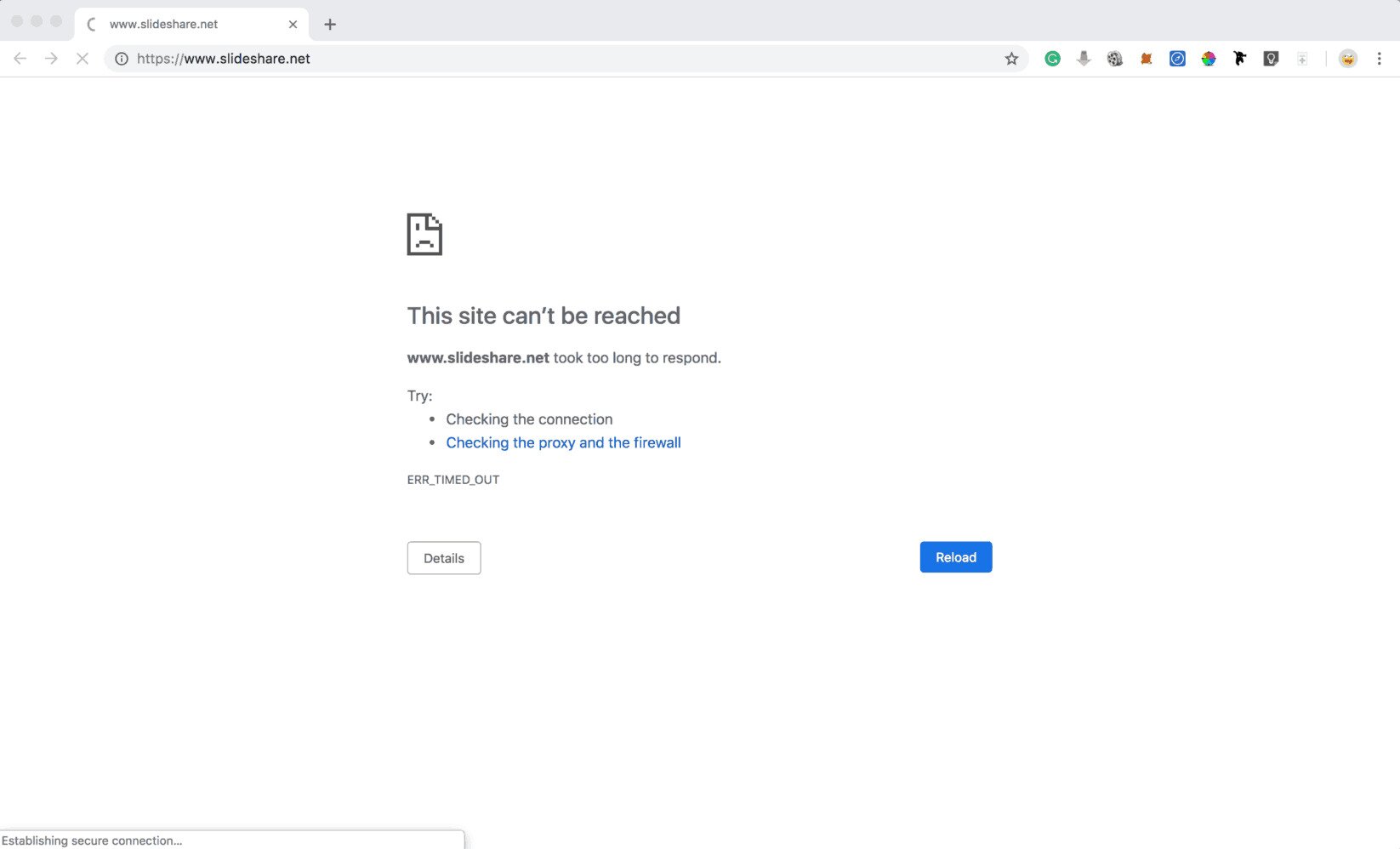Screenshot of a Browser Page Unable to Load

Description: This screenshot captures a browser page struggling to load the website www.slideshare.net. At the top, a gray bar hosts the browser's tabs and address bar. The affected tab is white and features the text "www.slideshare.net" along with a half-circle icon indicating the page is currently loading or unable to load. The address bar repeats the web address, flanked on the left by an 'X' and two arrows for navigation, and on the right by a star for bookmarking and other browser add-on icons.

Directly below the address bar, the main portion of the page displays an error message. A small page icon with a sad face sits at the top left of the message. The text reads, "This site can’t be reached," followed by "slideshare.net took too long to respond." Suggested troubleshooting steps include "Try checking the connection" and "Checking the proxy in the firewall." The error is identified as "ERR_TIMED_OUT." On the left side of the error message, there is a "Details" link, while on the right side, a "Reload" button remains highlighted, ready to attempt reloading the page.